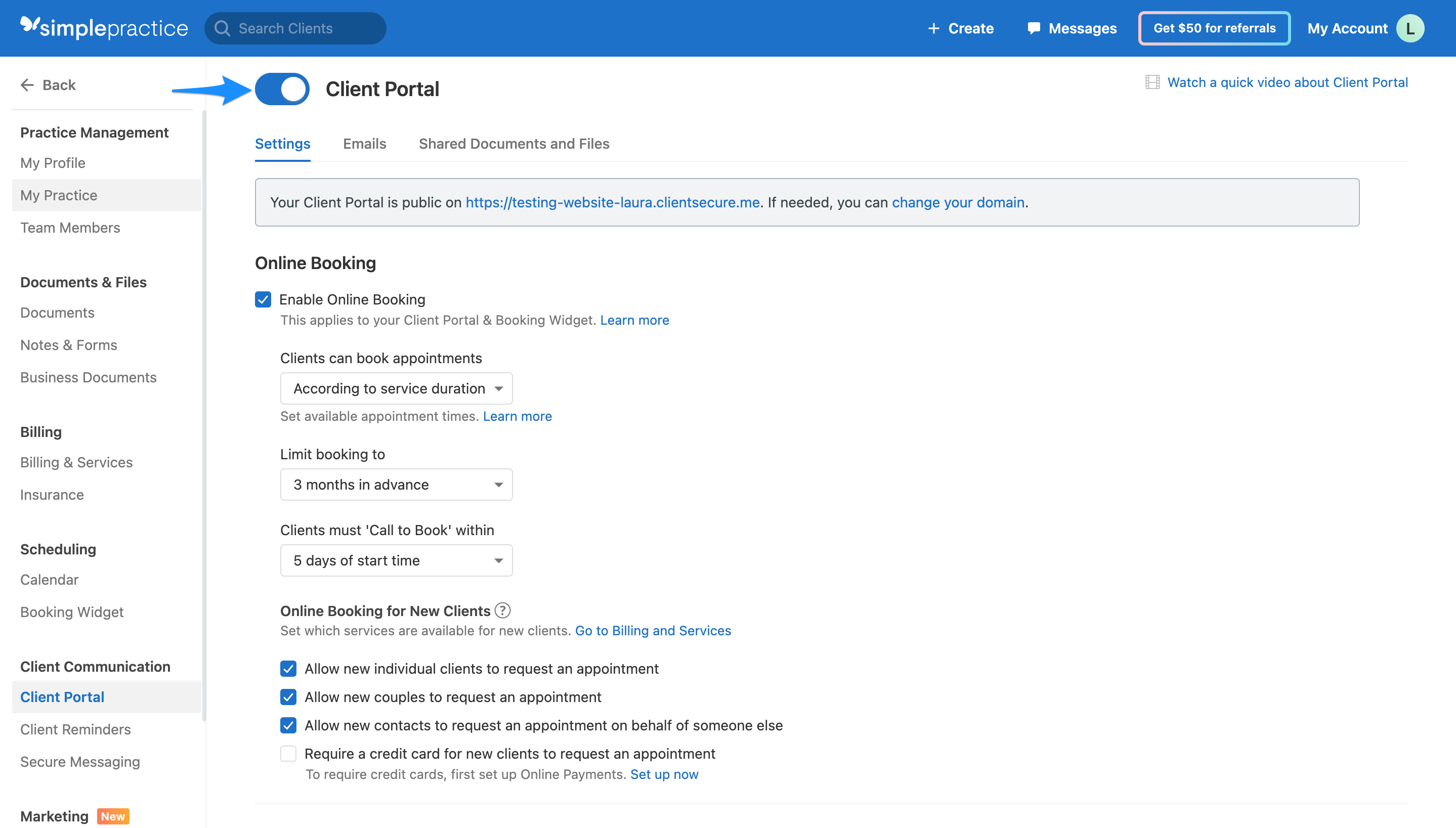A detailed screenshot on a laptop displays a webpage from "SimplePractice." At the top, a blue banner features a white butterfly icon beside the bolded word "Simple," followed by "Practice" in white letters. There is a search bar with a magnifying glass icon labeled "Search clients," a plus sign labeled "Create," and a messages icon. Further right, options for "$50 for referrals," "My account," and the user's profile bubble displaying an "L" are visible. Below, a prompt suggests watching a quick video about the client portal.

The user is currently on the "Client Portal" section, where a toggle button with an arrow is highlighted. Three subsections are outlined: Settings, Emails, and Shared Documents and Files, with the Settings tab active. The settings indicate "Your client portal is public on testing website Laura.clientsecure.me." Users can change the domain if needed and enable online booking, checked to allow clients to book appointments according to service duration, limited to three months in advance. Clients must call to book within five days of the start time.

Further settings show options to allow individual clients, couples, or contacts to request appointments on behalf of someone else, none of which require a credit card for new clients to book appointments. On the left-hand side, navigation options for practice management, documents and files, billing, scheduling, and client communication are listed.